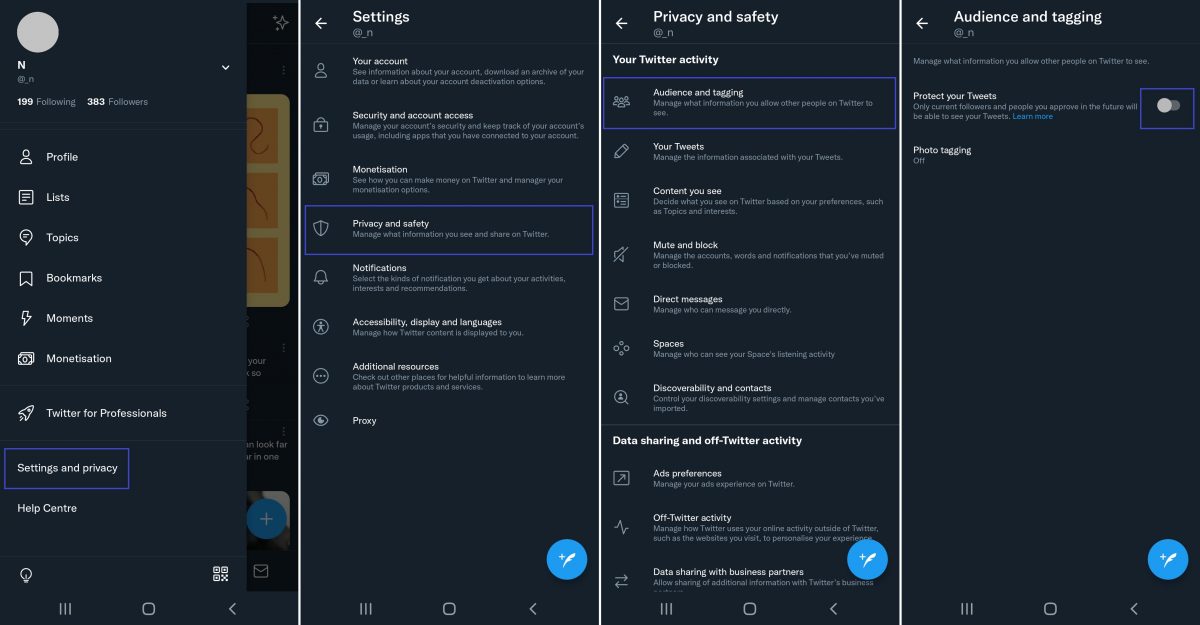This image presents a series of four screenshots from an Android phone, each illustrating different categories and settings within a social media app, likely Twitter. 

**First Screenshot (Top-Left):**
- Background: Dark gray.
- Upper Section: Displays a probable username in a white circle located in the upper left-hand corner, alongside follower and following counts.
- Categories Listed: Profile lists, Topics, Bookmarks, Moments, Monetization, and Twitter for Professionals, each accompanied by respective icons.
- Highlighted Section: "Settings and Privacy" outlined with a blue rectangle, followed by "Help Center".

**Second Screenshot (Top-Right):**
- Title: "Settings", indicated at the top with a small arrow.
- Options Displayed: Account, Security and Account Access, Monetization, Privacy and Settings, Notifications, Accessibility, Display and Languages, Additional Resources, and Proxy.
- Highlighted Section: "Privacy and Safety" outlined with a blue rectangle.

**Third Screenshot (Bottom-Left):**
- Title: "Privacy and Safety", marked with an arrow beside it.
- Options Displayed: Your Twitter Activity, Audience and Tagging, Your Tweets, Content You See, Mute and Block, Direct Messages, Spaces, Data Sharing and Off-Twitter Activity.
- Highlighted Section: "Audience and Tagging" outlined with a blue rectangle.

**Fourth Screenshot (Bottom-Right):**
- Title: "Audience and Tagging", with an arrow beside it.
- Options Displayed: Protect Your Tweets and Photo Tagging, including a toggle button for "Protect Your Tweets".
- Highlighted Section: "Protect Your Tweets" outlined with a blue rectangle.

Each of the three rightmost screenshots features a blue circle in the lower right-hand corner, possibly indicating a navigation or action button. The detailed categories and settings provide a thorough overview of the app's configuration options.